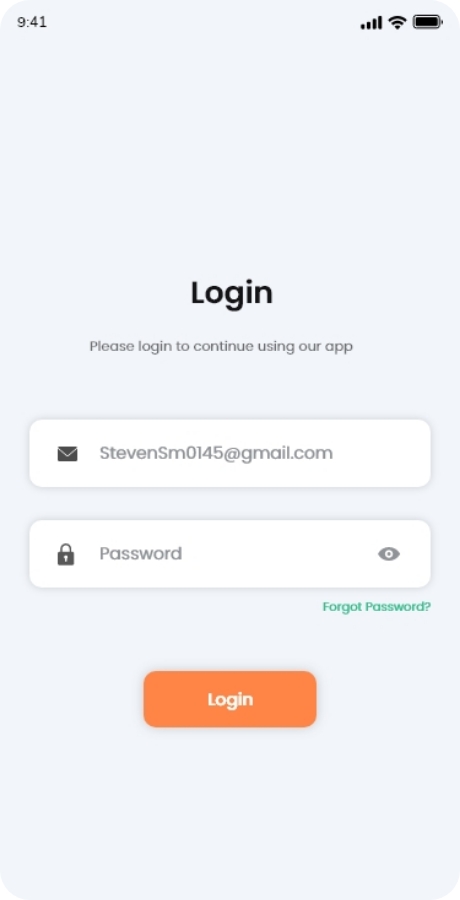This image captures a login page of a mobile application with a minimalistic interface set against a grayish-white background. 

At the top of the screen, the status bar displays at 9:41 (unspecified whether a.m. or p.m.) on the left. On the right, the signal strength indicators for both mobile data and Wi-Fi are visible alongside a fully charged battery icon. 

Centrally positioned, in bold black letters, the page title "Login" is prominently displayed. Directly below this, in smaller gray text, a centered subtext prompts: "Please log in to continue using our app."

The login section features two rectangular input fields outlined in gray. The first field, designated for the email, includes a male user icon and the pre-filled email address: "stephensmo145@gmail.com." The second field, intended for the password, includes a lock icon, the placeholder text "Password," and an eye icon on the right side for toggling password visibility.

Below the input fields, a green "Forgot password?" link is positioned on the right side.

At the very bottom of the page, an orange button with white lettering invites the user to "Login."